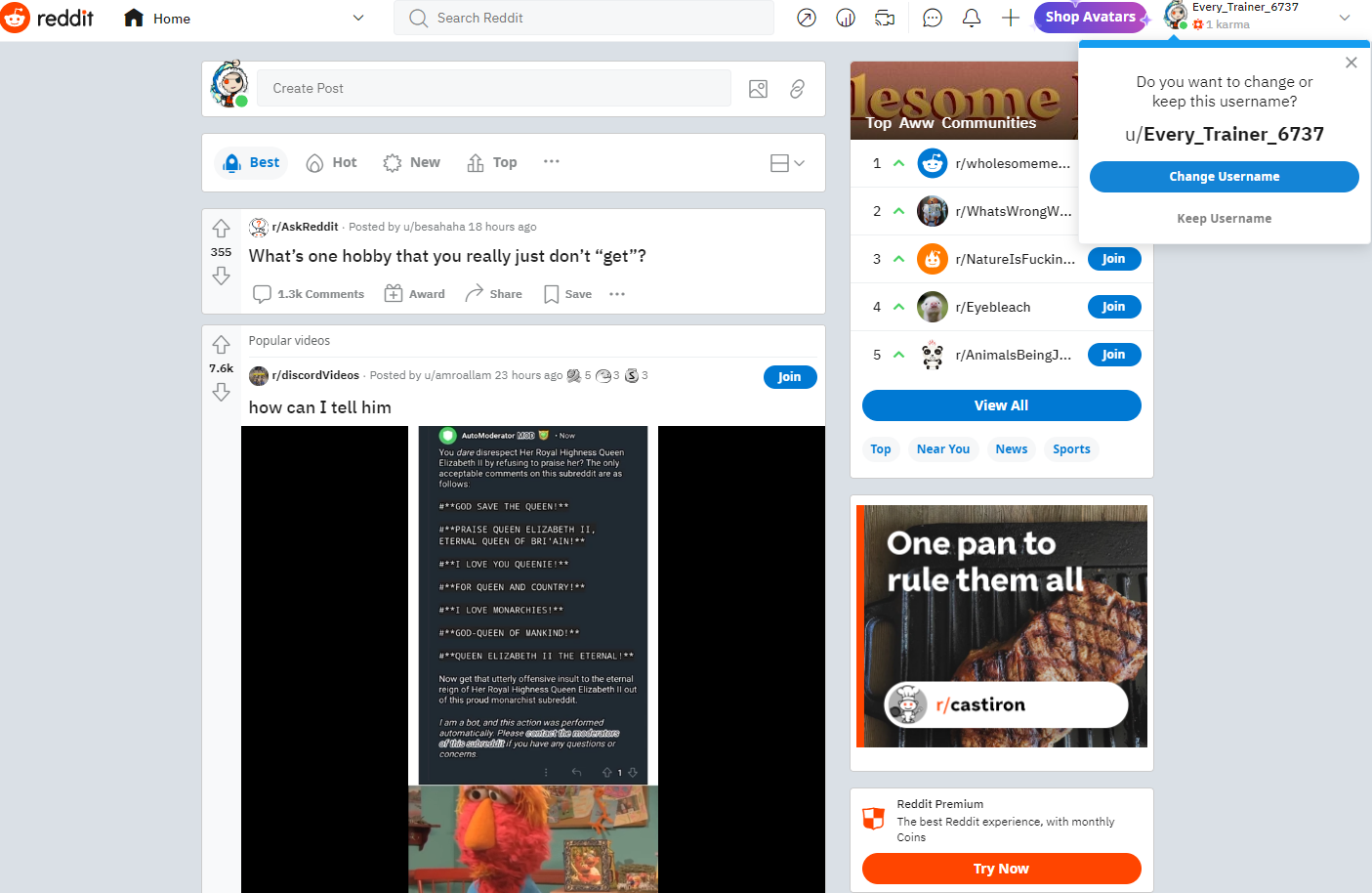**Image Caption: Detailed Reddit Homepage Overview**

The image captures the Reddit homepage, prominently featuring the Reddit logo on the left, followed by the text "Reddit" and the "Home" tab. In the center, there's a search bar labeled "Search Reddit." To the right of the search bar is a series of icons, possibly representing features such as a pop-out window, a film/video section, messages, notifications (bell icon), post creation (plus icon), and shop avatars.

Towards the top right, there's a section for user actions. It displays the current username, "every_trainer_6737," along with a blue button labeled "Change Username" and an "X" to close this option. There is also a gray "Keep Username" button.

In the middle of the page, there's a prompt to "Create Post" and filtering options labeled "Best," "Hot," "New," and "Top." Below, a post from r/AskReddit asks, "What's one hobby that you really just don't get?" This post has received 1,300 comments and 355 upvotes.

A subsequent section displays "Popular Videos" from r/videos, showing a post titled "How can I tell him? You dare disrespect her royal highness Queen Elizabeth II by refusing to praise her," emphasizing that the only acceptable comment on the subreddit is "God save the Queen, praise Queen Elizabeth II, eternal queen of Britannia, I love you Queenie, for Queen and country," followed by a user comment, "I love non-monarchies."